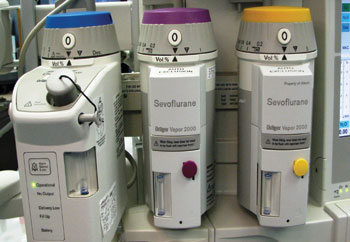This detailed indoor photograph captures three gray cylindrical medical devices lined up against a gray wall, resembling fire extinguishers in shape. Each device is topped with a distinct color: blue on the left, purple in the center, and yellow on the right. The panels are identified as being slightly lighter gray, and the two devices on the right are labeled "SEVOFLURANE." Their bases feature flat tops and rounded edges, with central white circles displaying the black number zero and an assortment of buttons and indicator lights. The leftmost device exhibits a slightly different configuration with a green light and what appears to be a vial inserted. Additionally, a black lead line with a circular attachment extends from this machine. Positioned to the right of these devices is a computer monitor, displaying an indiscernible software program due to the image's small and blurry nature. The scene includes some gray wires visible in the background, further emphasizing its medical or technical setting.